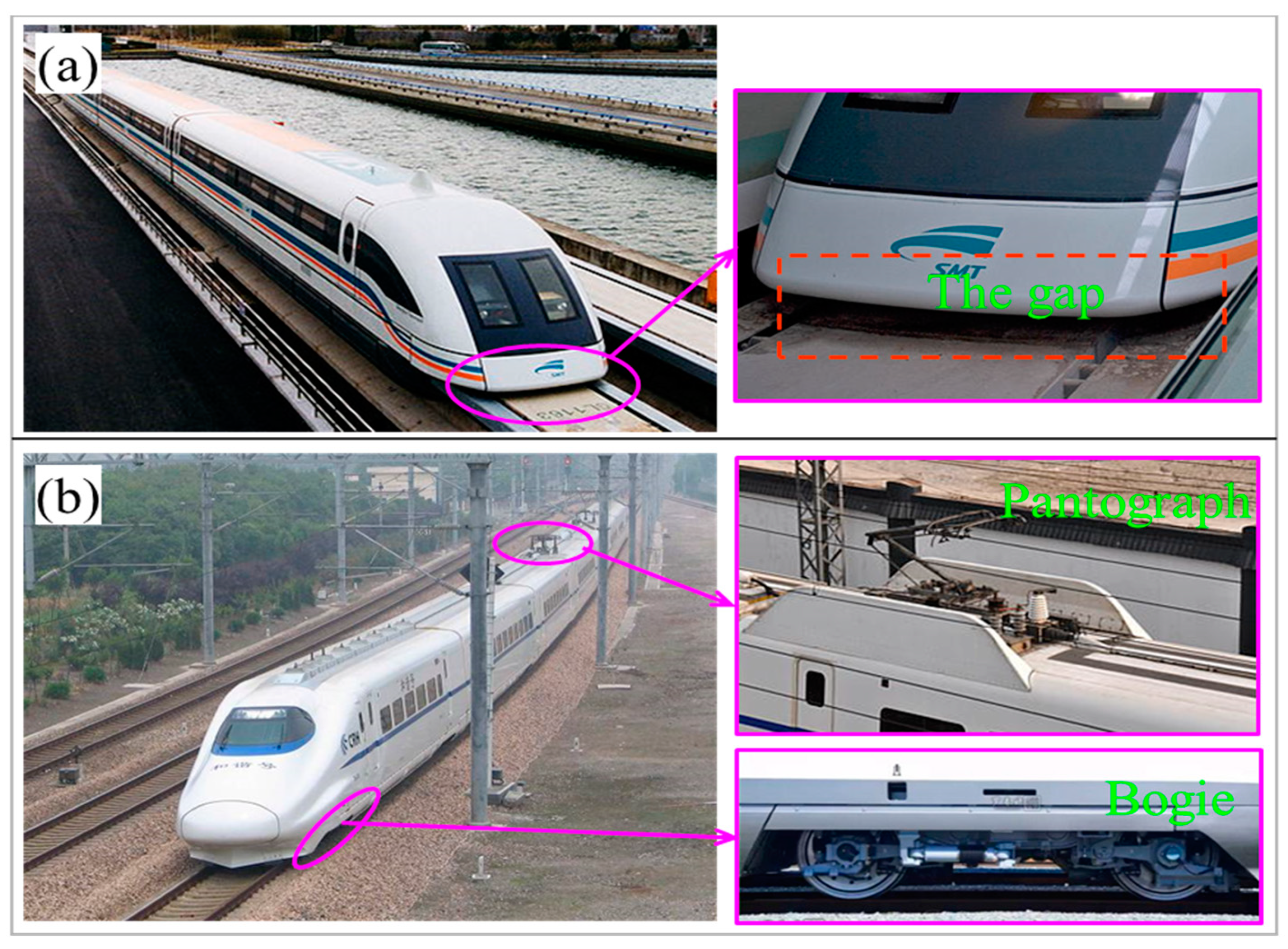The image is a collage of four detailed photographs of trains, organized within a large square and divided into labeled sections A and B. In the upper left corner (A), we see a high-speed, white train with orange and gray stripes, moving diagonally from the upper left to the lower right, adjacent to a body of water. This image is marked with a purple circle around the nose of the train, leading to the upper right corner, which showcases a close-up of the train's nose. Here, a broken orange line box highlights this area, labeled 'the gap' in green ink.

The lower half, labeled B, features another train, apparently a different type but also likely a passenger or speed train, traversing fields as it appears to be pulling into a station. The left image in section B shows a purple circle over the driver's side wheels and another purple circle and arrow indicating the pantograph on the third car's roof. The purple arrows guide viewers to the lower right image, which reveals a close-up of the wheels with the word 'bogie' in green font. The whole collage provides a comprehensive view of the various parts and functions of these trains.